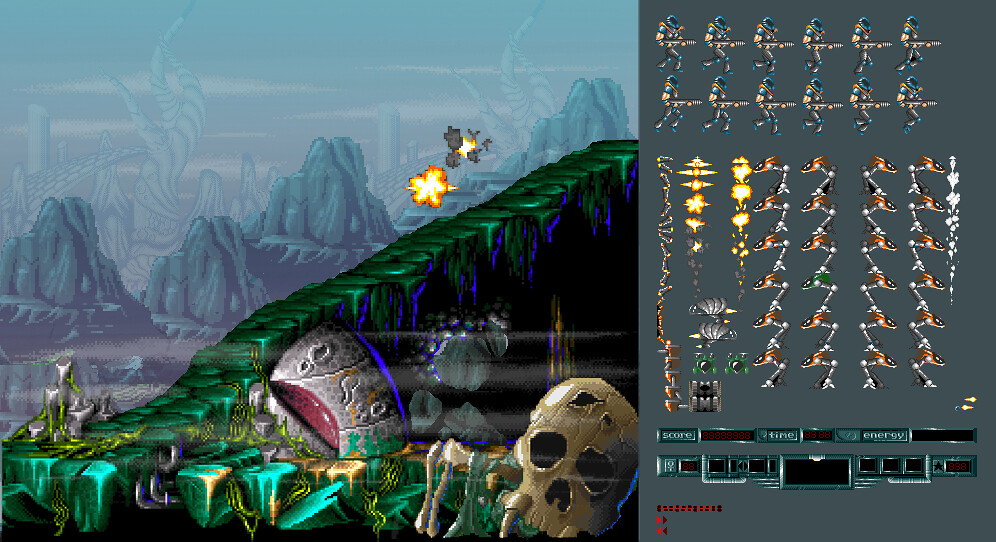This video game image is set against a blue background, interspersed with the ghostly, faded figures of large, wind-blown monster-like entities. In the midground, we see faint outlines of buildings, leading up to a range of darker blue-gray mountains. Prominently featured is a green structure which could be interpreted as either a bridge or an ascending staircase, extending towards the distant skyline.

Atop this structure, two explosions can be seen—one radiates hues of orange and yellow, while the other is shrouded in gray. Descending to the bottom of the image, a series of white pillars emerges from the ground, culminating in a large, ominous skull with gaping eye and nose cavities.

Over this skull looms a ghostly image of dangling legs, suggesting a spectral figure seated on the edge of the bridge-like structure. Adding to the eerie scene, near the bottom right, there is a mysterious entity that might either be a ship or a boat with a dragging feature, or a fearsome monster brandishing a large, menacing red mouth.